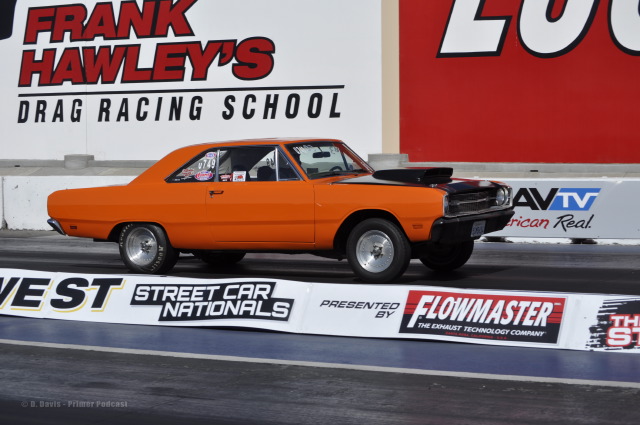In the image, a striking, pumpkin-orange muscle car from the 60s or 70s with a prominent black hood and a large exhaust is the central focus. The car, adorned with decals on its windows, is positioned directly in the middle of the scene on an oil-slicked drag strip. The setting appears to be part of a drag racing school event, featuring several prominent signs. A banner near the bottom center reads, "Street Car Nationals presented by Flowmaster," the exhaust technology company. To the left, a sign reads "Frank Hawley's Drag Racing School" in white and red with a black underline. The background is filled with various advertising signs, including a predominantly red one showing just the letters "LOL." The overall color palette includes shades of gray, black, dark blue, white, red, orange, silver, and maroon, enhancing the vivid atmosphere indicative of a high-energy car show or racing event.